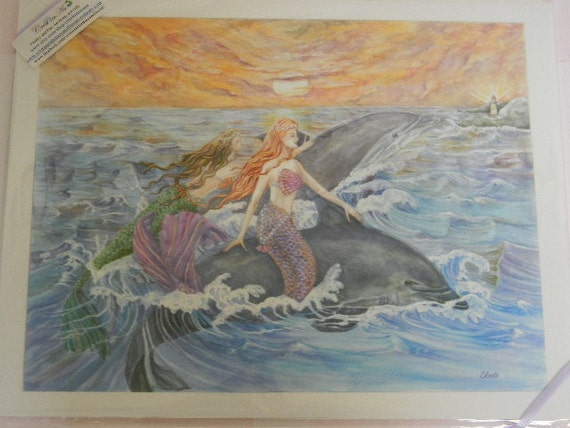This image features a vibrant illustration, possibly a watercolor painting or colored pencil drawing, encased in a clear yellow cellophane wrapper and adorned with a ribbon at the corner. A small, unreadable sticker, likely containing the title and artist’s contact information, is affixed to the cellophane. The artwork itself depicts an enchanting scene of two mermaids riding dolphins during a sunset. One mermaid, with orangish hair and a pink tail, sits sidesaddle on a dolphin partially submerged in water. The second mermaid, with brown hair and a green tail, is grasping the dorsal fin of another dolphin as it leaps from the ocean, creating splashing waves. The pastel colors of the mermaids contrast beautifully with the purple and blue hues of the ocean, while the sky is bathed in a warm golden glow of the setting sun. In the distance, a lighthouse emits a soft shine, adding an element of serene guidance to the fantastical marine tableau. The artwork appears to be set against a poster board backing, suggesting it might be an item available for sale, possibly on a platform like eBay.